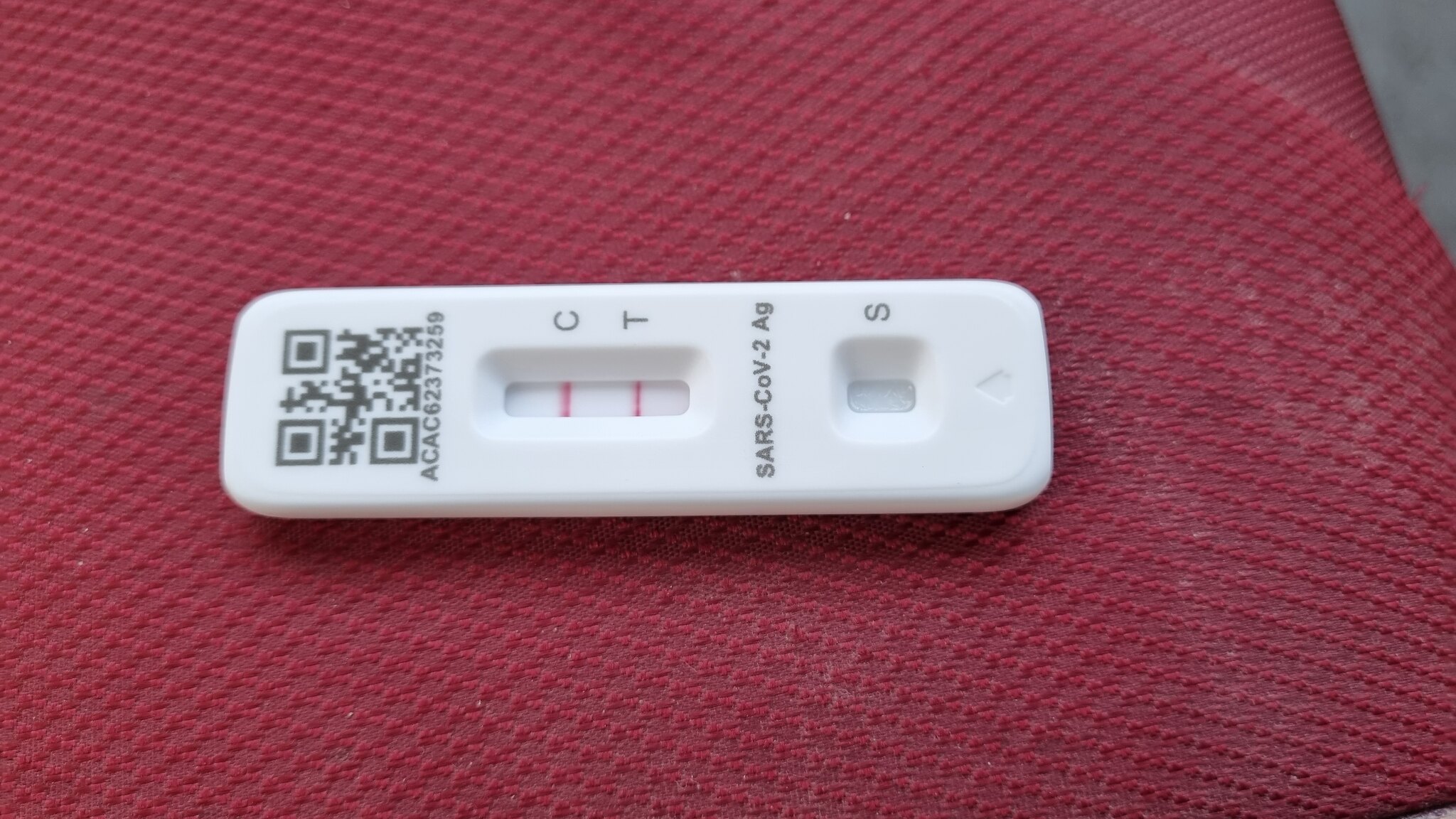The image captures a simple yet detailed scene centered around a thermometer placed on a red pillow with a rough, textured design featuring diagonal stitches. The red pillow occupies about 95% of the background, while a small section at the top right reveals a grey background. The pillow shows some faint white stains on the right side. The thermometer is positioned sideways, turned counterclockwise, with a black QR code visible on its left side. In the center of the thermometer, a small rectangular display on a white background shows two red lines, labeled with "C" for control and "T" for test. On the far right of the thermometer's display, there is a small box marked with the letter "S." Below this, towards the bottom-middle of the thermometer, the text "SARS-COV-2 AG" is printed.